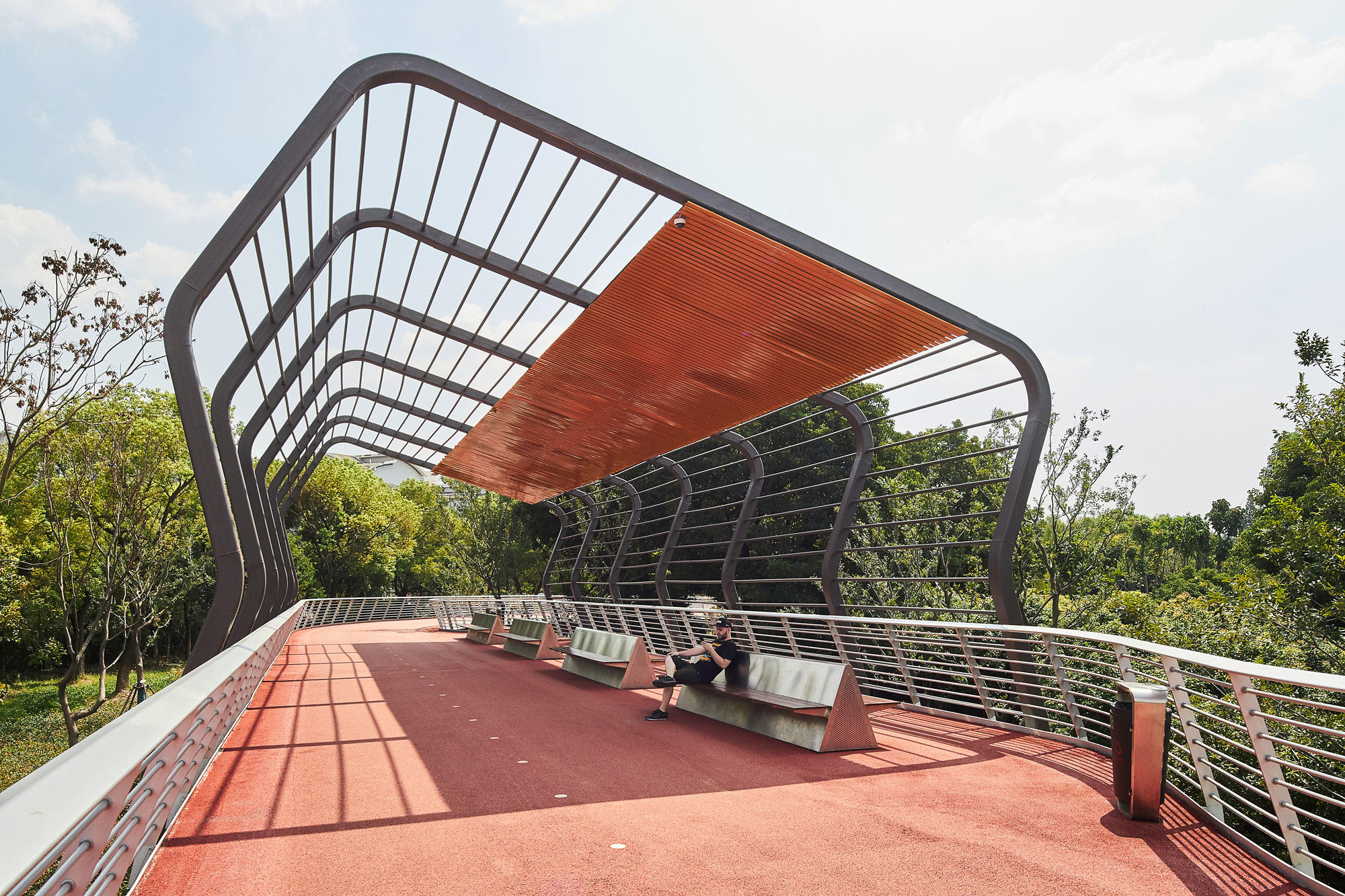In this detailed photograph, a unique and modern walking bridge is captured on a bright sunny day with lightly cloudy skies. The bridge features a reddish-brown or orange pavement and is surrounded by sleek, silver metal railings that curve gracefully upwards, forming a trellis-like structure that arches overhead. The top of the trellis boasts a distinct copper design, adding an artistic touch while providing shade. Four contemporary metal benches line the bridge, with a single man in a black t-shirt, shorts, and a cap sitting on one of them. The surrounding landscape is lush with green trees, lending a serene ambiance to this inviting, ship-shaped pedestrian pathway.